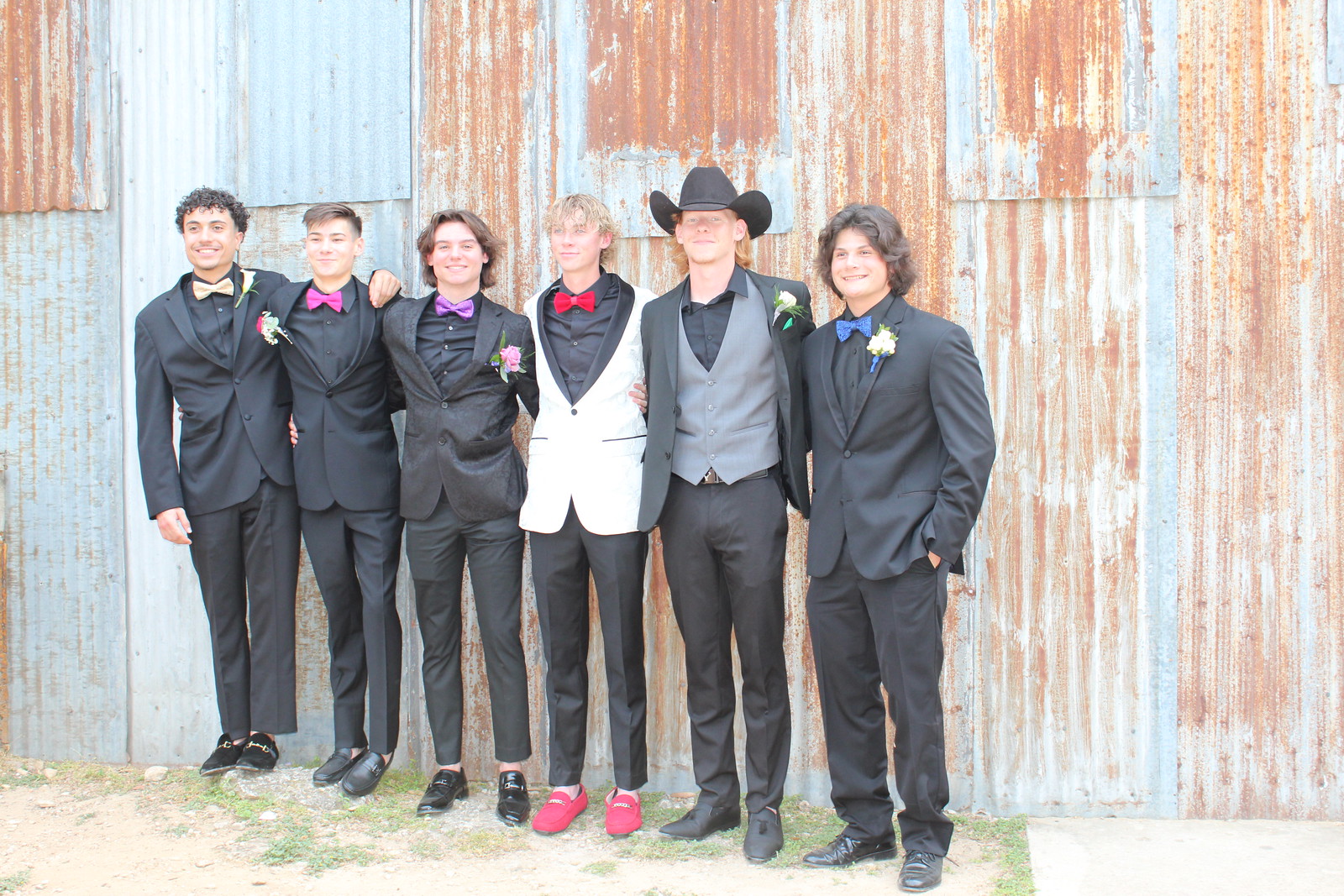A group of six young men, likely high school age and preparing for a formal dance, are posing in front of a corrugated tin wall that alternates between gray and rust colors with visible stripes. They are all dressed in suits with gray pants, and all but one are wearing gray jackets; the exception is the young man in the center, who sports a white jacket. All but one are donning bow ties: the man on the far left has a tan bow tie, followed by a pink, purple, and red bow tie in sequence. The last individual on the right wears a blue bow tie. The one who stands out is the fourth individual from the left, who wears a black cowboy hat and forgoes a bow tie in favor of a collared shirt and vest. Four of them have flowers pinned to their lapels, adding a touch of elegance to their attire. They are positioned outdoors, likely in a rural or country setting, enhancing the informal yet polished vibe of the gathering.